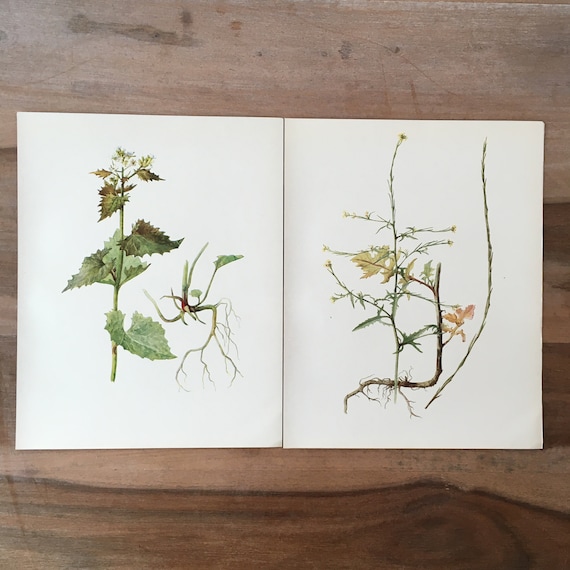This image showcases two pieces of paper, seemingly extracted from a sketchbook, placed side by side on a wooden surface, possibly a table or floor, with a faint crease indicating they are separate sheets. Both pieces feature intricate watercolor illustrations that hint at a woodland theme. 

The left piece displays a delicate stem adorned with green leaves, tapering off into sparse, brown-tinted leaves near the top. Intriguingly, it also depicts a whimsical figure resembling a "root fairy" with what appears to be a combination of roots and a stem forming a body with an arm, exuding a magical, nature-inspired aura.

The right piece complements the first with thin, vine-like branches bearing clusters of smaller, orangey-yellow leaves and buds. These branches are densely adorned, contrasting the sparser foliage of the left piece. Both artworks share a cohesive artistic style, suggesting they are the creations of the same artist.